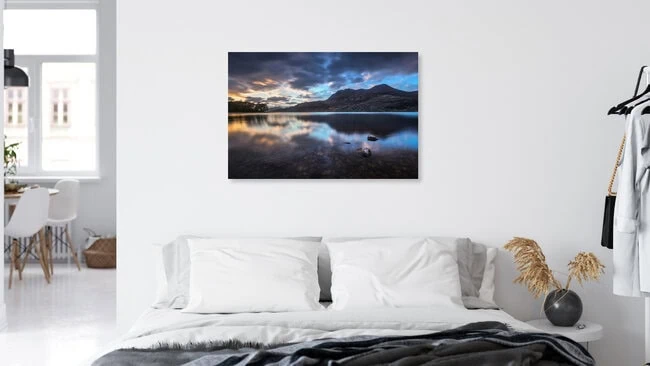This horizontally aligned photograph captures a modern, open-floor-plan apartment with seamless transitions between spaces. The image predominantly showcases a minimalist bedroom on the right side, which takes up about four-fifths of the frame. The walls and floor are immaculately white, lending a crisp, clean atmosphere to the area. The understated bedroom features a double bed with a slightly rumpled, dark gray blanket draped over its lower half, topped with white pillows. Propped up against the wall behind the bed, the headboard may be gray, offering slight color contrast. 

Above the bed, a striking piece of art draws attention; it depicts a serene outdoor scene with a mountain range reflected in a still lake. The sky in the artwork shows transitions from blue to shades of gray and peach, suggesting an early evening setting. Next to the bed stands a small, white circular end table that holds a black vase containing dried, decorative fronds in light brown hues.

To the right of the bed is an open area dedicated to storage, featuring a white clothes rack. This rack is meticulously arranged with neat, white garments and a black purse with a gold chain, hanging from black hangers.

In the background, the bedroom opens up into what appears to be an informal dining area or kitchen. This space is marked by a round table with a wooden top and white base. Surrounding the table are minimalist, white armless chairs with brown wooden legs, evoking a 70s aesthetic. On the floor near the table stands a white basket and a heater or radiator, possibly hinting at the apartment's functional elements. The top of the table has some debris, adding a faint touch of lived-in realness.

A horizontally aligned rectangular window comprises three panes – an upper horizontal pane over two vertical ones. Through the window, we see another building with white-framed six-paned windows, amplifying the sense of openness. A house plant, possibly a spider plant, sits on the windowsill, enhancing the homely ambiance.

The pervasive use of white throughout the apartment, the fine lines, and modern furnishings, all contribute to an airy, contemporary aesthetic, possibly resembling an Ikea advertisement from recent years.